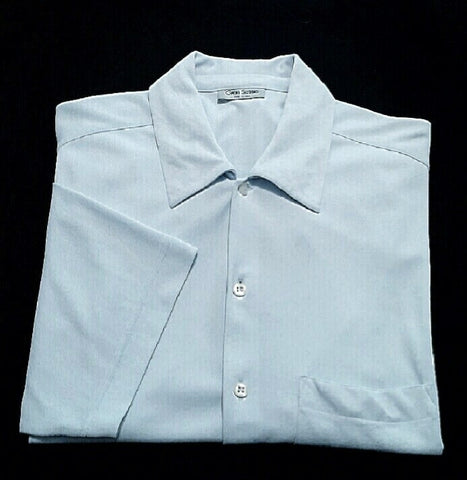This is a detailed color photograph of a very light blue shirt, neatly folded against a black background. The shirt features a small, pressed collar and is buttoned down the front, showcasing three shiny white buttons. It has short sleeves, with the right sleeve folded forward for display, and a pocket on the left side. The fabric appears to have very faint pinstripes, adding subtle texture to the shirt. This shirt, possibly a casual or pajama style, could be suitable for a work setting. Its presentation suggests it might be featured in a catalog, highlighting its polished and formal appearance while emphasizing its neat folding and overall tidiness.